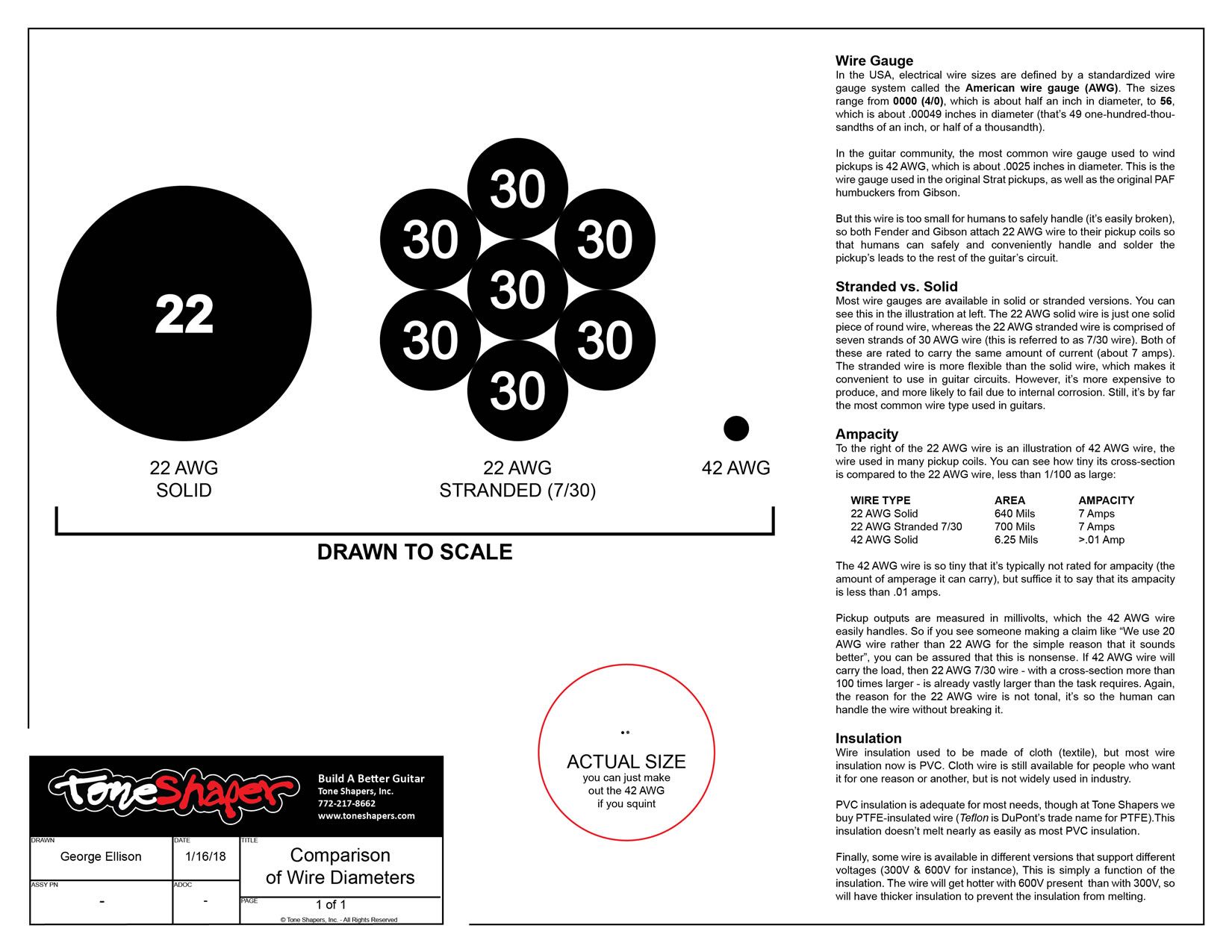This scanned image is a detailed chart focused on wire specifications, emphasizing their application in guitar building. The rectangular image has a thin black border, and it's packed with text and diagrams. At the top left, a prominent black circle features the white number "22" and is labeled as "22 AWG Solid," indicating solid wire. Adjacent to this, seven black circles arranged in a flower pattern also contain the number "30," illustrating a stranded wire configuration. Near these diagrams, there's another tiny dot labeled "42 AWG," with an adjacent red circle marked "actual size".

In the bottom left corner, the text reads "Build a Better Guitar" alongside branding for "Tone Shaper," including a phone number and a website. Additionally, there's a comparison of wire diameters labeled beneath the diagrams. The right side of the image hosts multiple paragraphs under the heading "Wire Gauge," delving into details like stranded versus solid wires, ampacity, wire type, and insulation characteristics. Overall, the document merges both diagrams and descriptive text to provide a comprehensive overview of wire gauges, emphasizing their relevance to enhancing guitar tones.